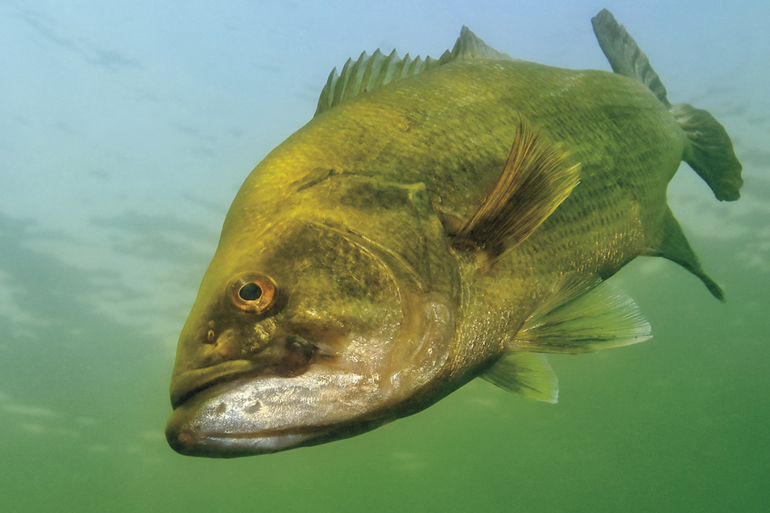The image portrays a large fish, possibly a bass, underwater. The fish, captured in a curved, slanted motion as if swimming downward towards the left side of the picture, dominates the center. Its body showcases a blend of green and yellow hues, with a silver bottom jaw and golden eyes with black irises. The fish has multiple visible fins, including those on its back and tail, with the tips appearing yellowish-green. The water background transitions from bluish near the surface to a greener shade towards the bottom, enhancing the overall aquatic ambiance. The fish's mouth is closed, and its detailed features are sharply defined, including the scales and the underside, creating a vivid and dynamic underwater scene.